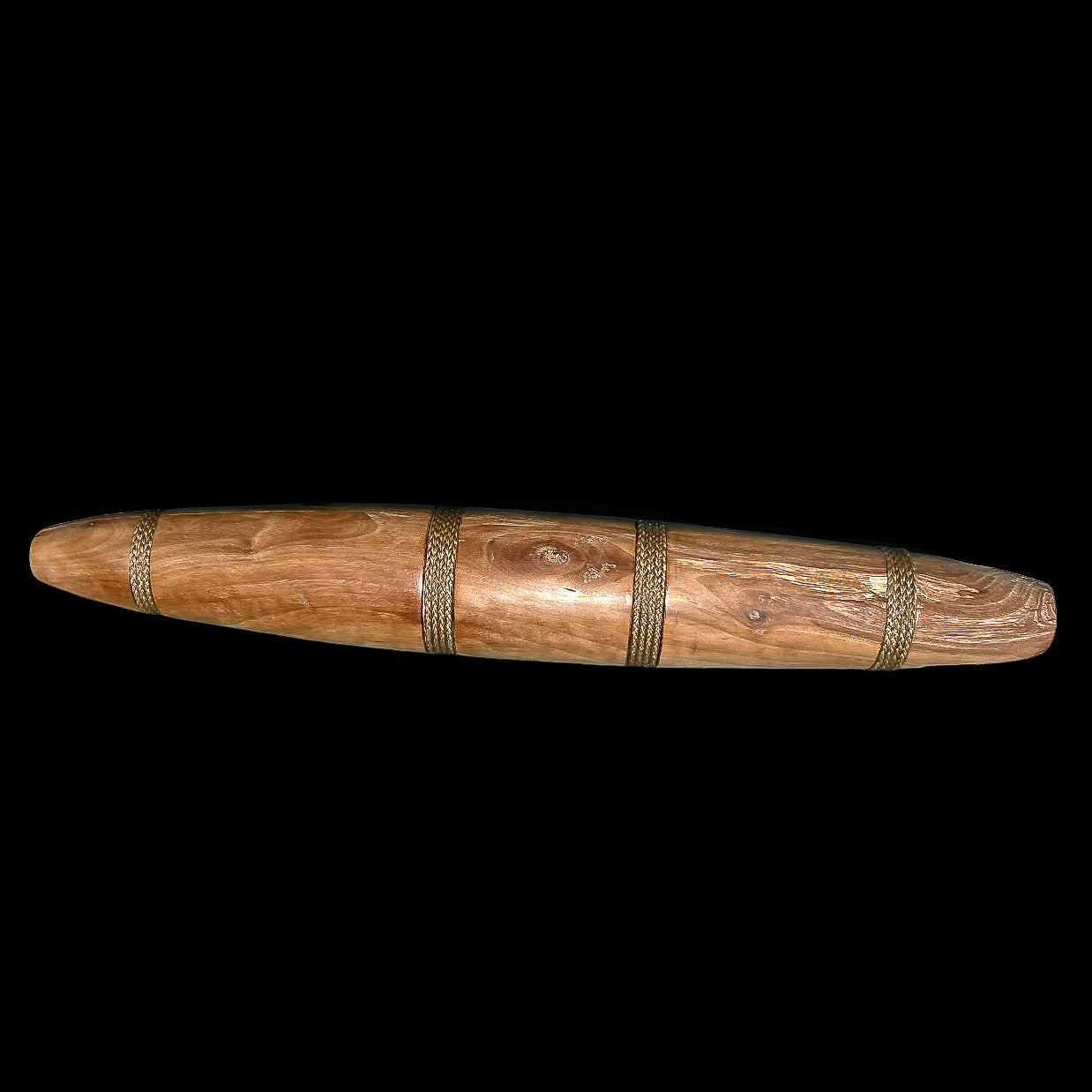The image depicts an intriguing, close-up view of an elongated, cigar-shaped wooden object set against a stark black background. The wood exhibits distinct texture and visible grain lines, suggesting it is old and dried out. The object features four intricately detailed bronze-colored bands, possibly made of fabric, rope, or twine, wrapping around it. The wood has a medium yellowish-brown tone, with certain areas showing varying shades and signs of wear, particularly at one end. The bands are likely functional, perhaps serving to keep the object, which seems to be composed of two separable pieces, securely closed. The worn texture contrasts with the lustrous bands, enhancing the object's unique and antique appearance.